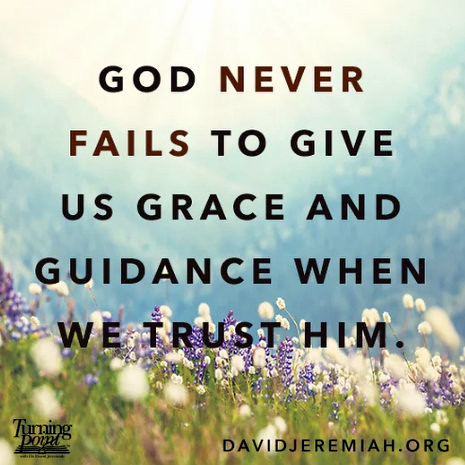The image is an inspirational photo featuring a field of green grass dotted with purple and white flowers in the forefront. The background showcases a majestic landscape of multiple mountain slopes under a partly cloudy sky, with the sun peeking over the top. Overlaid on the photograph is a quote in bold black text that reads, "God never fails to give us grace and guidance when we trust Him." Positioned in the bottom corners, in black text, are two additional elements: on the right, the website address "DavidJeremiah.org," and on the left, the logo of an open book with the text "Turning Point" beneath it, accompanied by smaller, unreadable text. The overall composition and message aim to provide spiritual encouragement.